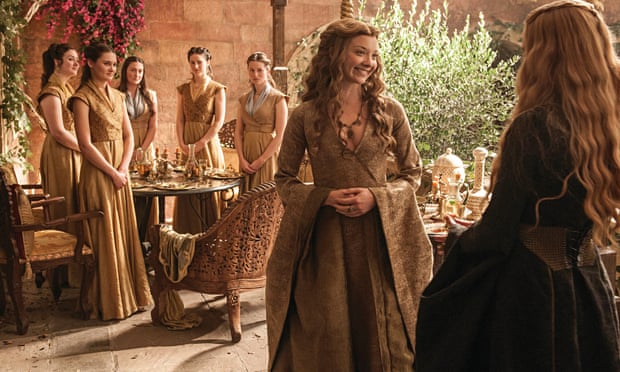The photo captures a unique, vintage-style scene with several women dressed in intricate Game of Thrones-inspired gowns, evocative of a Renaissance Festival. The background features a brown wall with some plants suggesting a courtyard setting. In the center and foreground, two women stand out prominently. The woman in the middle has wavy, long brown hair, is smiling, and is dressed in a long, flowing, deep V-neck goldish-brown gown with wide, extended sleeves. She clasps her hands in front of her and wears a necklace. To her right is another woman with similarly wavy, long brown hair, wearing a black gown cinched with a white belt, her back partially turned to the camera.

To the left, a group of five women stands around a round table with elaborately carved wooden chairs. Their hands are also clasped in front of them. They are uniformly dressed in long, light-brown sleeveless gowns that reach the floor, and all of them have long brown hair cascading below their shoulders. The table is adorned with what appear to be wine glasses and other items, completing the detailed and atmospheric tableau.